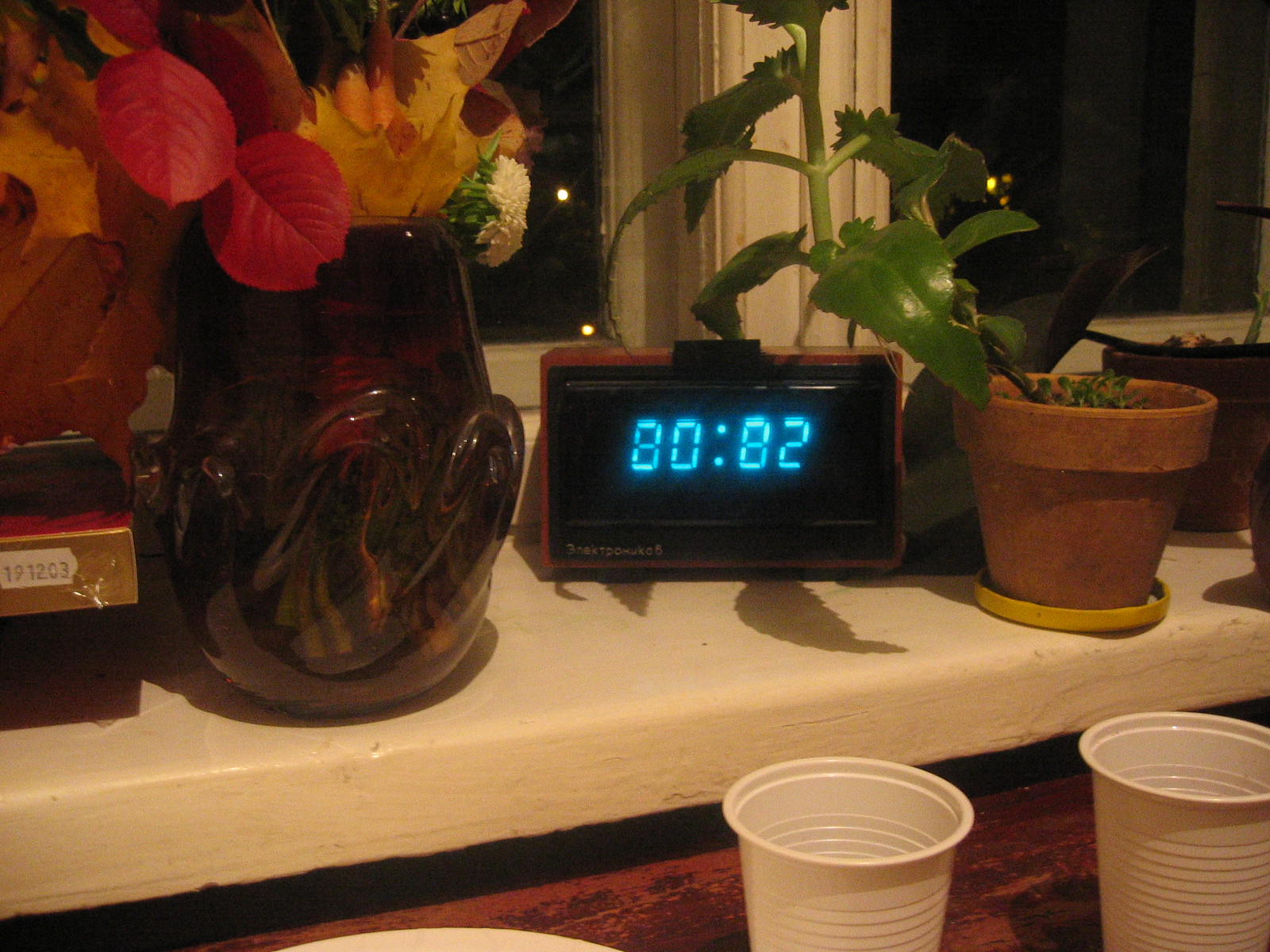The photograph captures a close-up view of a white window ledge adorned with various objects, set against the backdrop of white-framed windows. Centrally positioned on the ledge is a black rectangular digital clock displaying the numbers "80:82" in bright blue, indicating it’s malfunctioning. The clock is framed by a brown border. To the left of the clock stands a glass vase with a brown tint, decorated with rooster or mushroom patterns, containing artificial flowers in shades of reddish-orange and white. To the right sits a small brown ceramic pot with a green plant, characterized by a large stem and lush leaves. In the foreground, there is a brown table with two white plastic cups visible atop it.